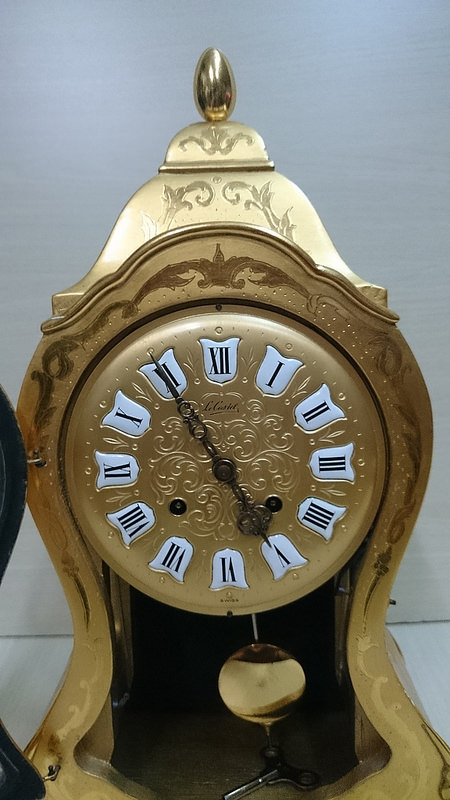The image showcases a close-up photograph of an antique-style, gold-finished clock with intricate Victorian-era detailing. The clock features a polished, egg-shaped top and an hourglass-like, wide midsection. The clock's round face displays black Roman numerals set against a white background adorned with tulip or daffodil motifs, ranging from I to XII. The hour and minute hands are black, positioned at five minutes to five. Below the clock face, within an open enclosure, sits a key for winding the clock, indicative of its old-fashioned, mechanical operation. This enclosure likely also houses a pendulum, though not clearly visible. The clock, equipped with a hinged door for accessing its interior, rests on a white surface in front of a light blue backdrop. Intricate sketchings embellish its top section, adding to the antique's ornate design, suggesting it's a valuable collectible. To the left, there is a partly visible object adding context to the setting.